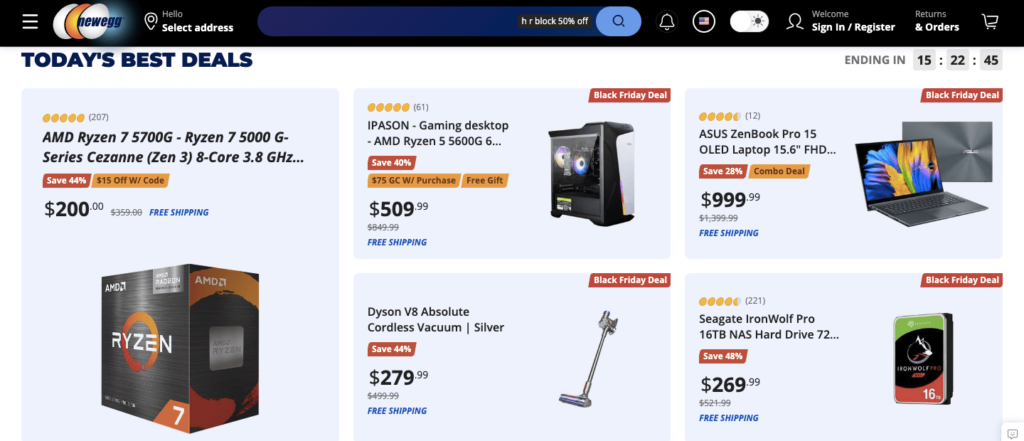An image promoting "Today's Best Deals" features various products presented in a neatly organized and visually appealing layout. In the top-left corner, you'll see three horizontal bars acting as the menu icon. Directly below, there's an offer for a Ryzen 5 5000G series processor priced at $200. Adjacent to it on the right is an image of a gaming desktop equipped with AMD Ryzen, priced at $509. To the right of that, there is a sleek ZenBook laptop, showcased with a price tag of $999.99. 

Moving towards the bottom-center of the image, a Dyson Absolute Cordless Vacuum in silver is displayed for $279. Positioned to the right of the vacuum is a Seagate IronWolf Pro 16TB hard drive. In the top-right corner, an icon for orders, a shopping cart, and options to sign in or register can be found alongside an American flag.

The bottom-right corner includes a clickable area that opens a chat window for customer support. The majority of the background features light blue boxed sections for each product image. Prominently placed at the top is a black search bar, accompanied by a blue circle containing a magnifying glass icon for search functionality.